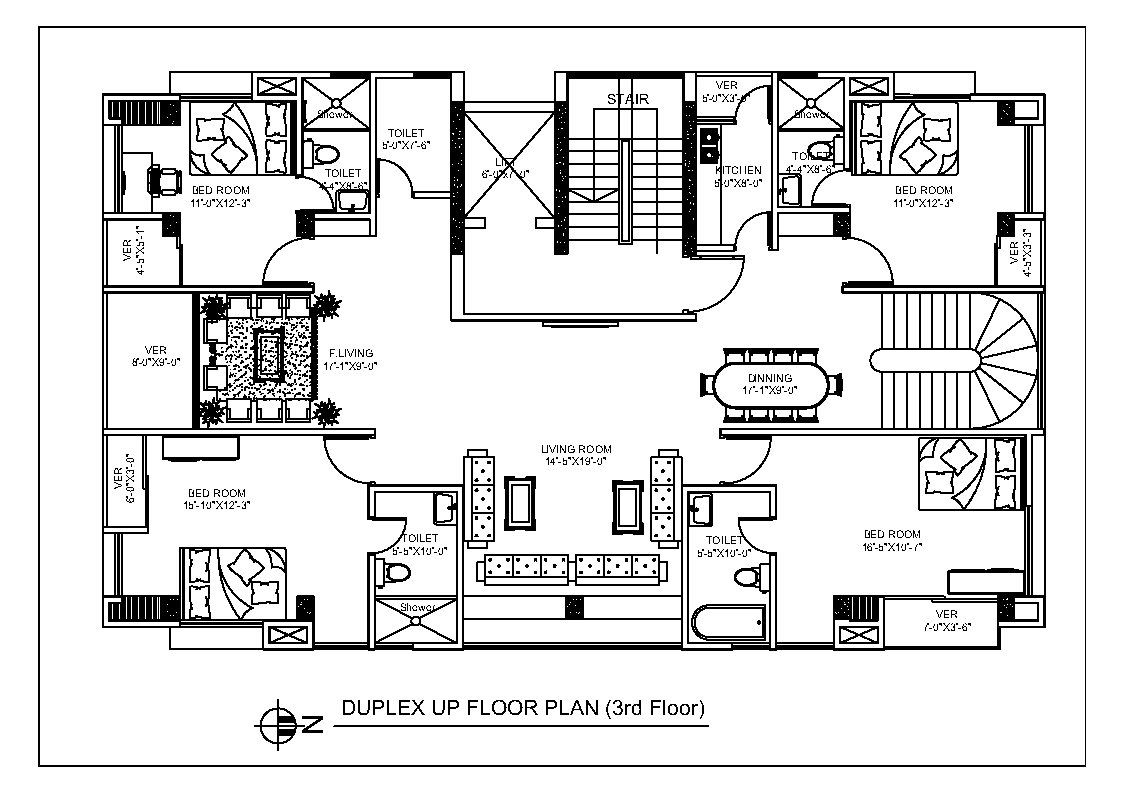This is a detailed and intricate drawing of the third floor of a duplex floor plan, complete with directional designations for north, south, east, and west. The layout features four bedrooms, each situated in the corners of the design, providing ample privacy and space. There are four bath areas: one with a full bath and the others equipped with showers. The living area is centralized, complemented by a spacious, full dining table and a cozy living room located at the bottom section of the plan. 

A remarkably elaborate stairway is positioned on the far right, leading to different levels, and an additional stairway is sketched at a lower level for convenience. The far left of the plan showcases an inviting outdoor veranda, perfect for relaxing and entertaining. Other notable features include ample closet space and what appears to be an outdoor patio area, enhancing the luxurious feel of the design. The overall layout is a high-end, sophisticated representation of a third floor in a duplex, meticulously detailed and thoughtfully designed.